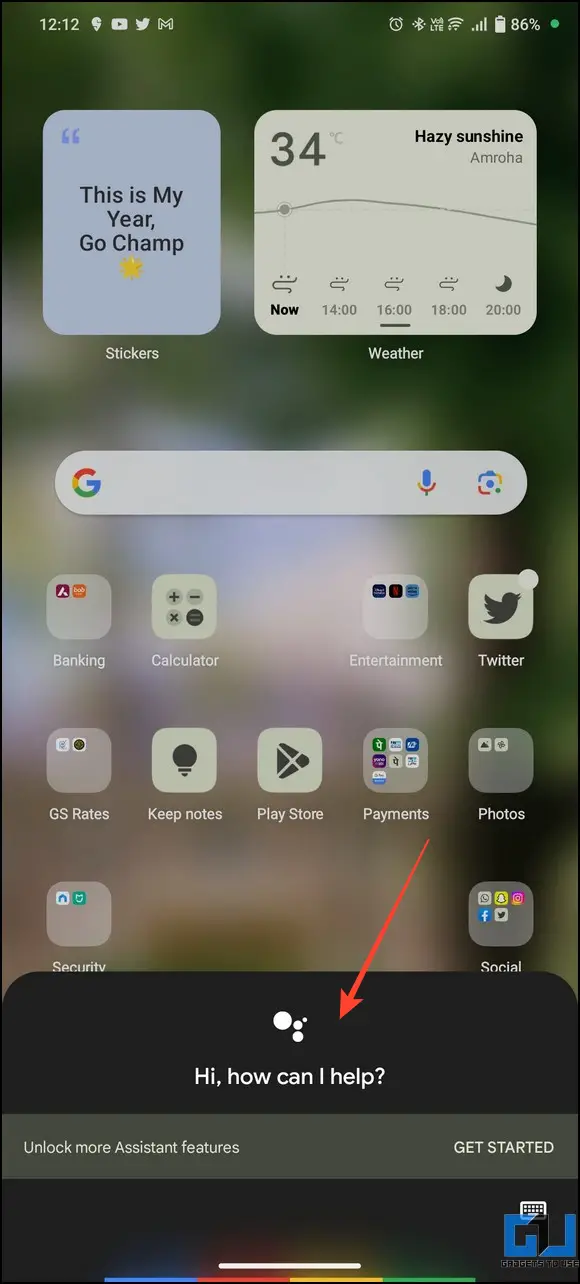This screenshot from a smartphone showcases a meticulously organized home screen with a blurred outdoor background. A faint green hue runs along the right edge of the screen and stretches across the top, with a earthy brown tone at the bottom, suggestive of ground. On the left side of the status bar, the display shows the time, location icon, YouTube icon, Twitter icon, and Google Mail icon. On the right side, a green circle is present, followed by a white background displaying an 86% battery life, full internet and Wi-Fi signals, an LTE indicator, a Bluetooth symbol, and an alarm clock icon.

Moving down to the main interface, the left section features a blue and white square with black text inside reading "This is my next," followed by "You're a common," and "Go champ." Below it, there’s a yellow circle labeled "Stickers" in white text, with the sticker being slightly larger than a regular icon. To the right is a larger square with a whitish-gray background. It contains big black lettering with the number "34" in the top right corner and an umbrella icon, indicating "hazy shine," with a black line dividing the section. Below this, a timeline with "now," "1400," "1600," "1800," and "20" markers appears, labeled "weather" in white text.

A search bar stretching horizontally occupies the space below, featuring the Google icon on the left, a microphone icon, and a photo icon. Underneath, the app section is neatly laid out with four apps in the top row: Banking, Calculator, Entertainment, and Twitter, leaving a blank space in the center. The second row lists five apps, from left to right: GS Rates, Keep Notes, Play Store, Payments (highlighted in white), and Photos. Under the Payments app, another prompt reads, "How can I help you?" near the bottom of the screen.

Further down, one icon on the left says "Security" and another on the right says "Social." A prominent black bar just above the bottom reads, "How can I help you?" A gray tab below it states, "Unlock more assistant features," with "Get started" highlighted on the right end.

This detailed illustration encapsulates the organized structure and diverse functionalities available on this smartphone’s interface.